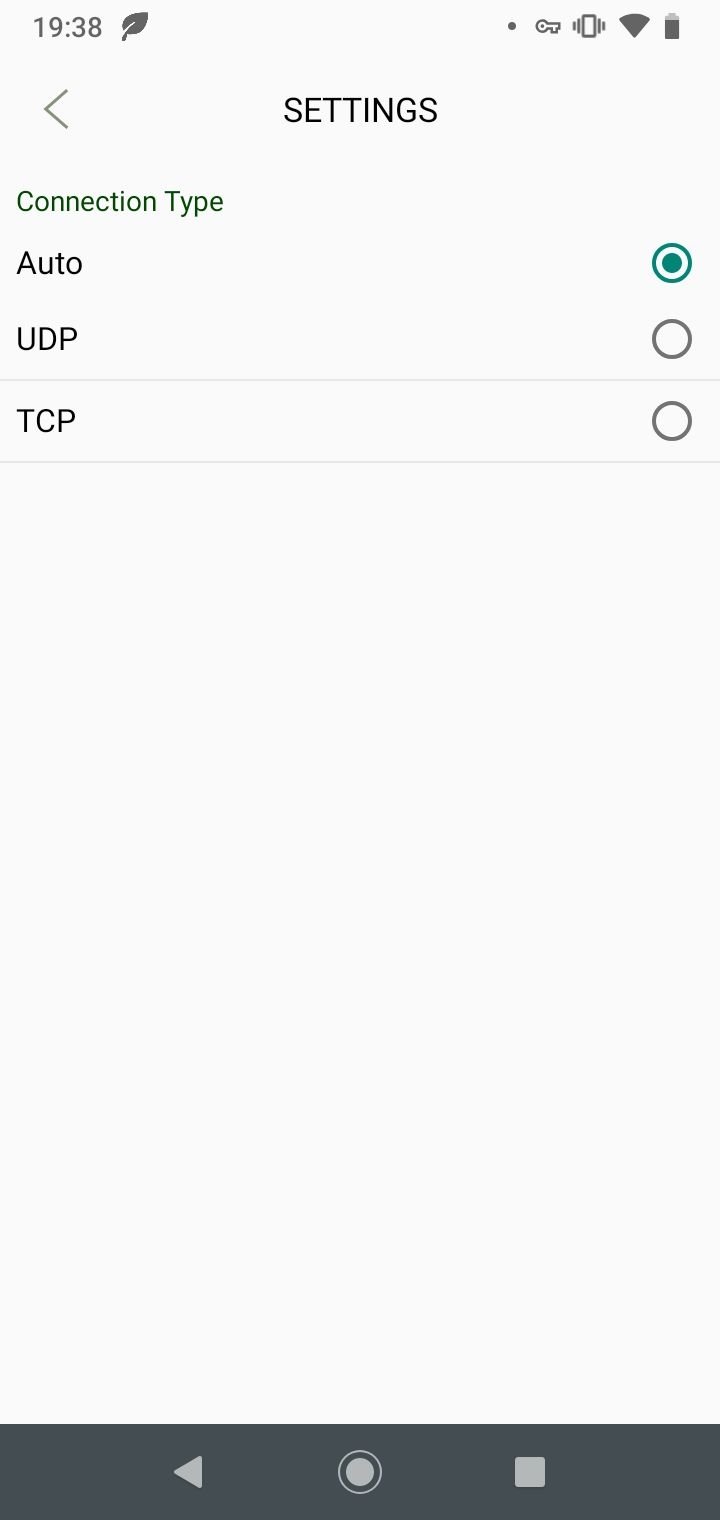The image captures the settings options menu of either an application or a website, presented on a predominantly white background with a dark grey section occupying the bottom 5-10% of the screen. At the top of the interface, in grey text, the number "1938" is displayed alongside a leaf icon for visual distinction. Adjacent to this, there is a sequence of status icons: a dot, a key icon, a vibrate icon, a fully-filled WiFi signal icon, and a battery icon indicating approximately 90% charge.

Directly beneath this header, aligned to the left, is a grey left-pointing button, and to the right of this button, in black text, is the label "Settings." Below this, on the left side of the layout, the term "Connection Type" is labeled in dark green text.

The menu provides three radio buttons for selecting the connection type, listed vertically as "Auto," "UDP," and "TCP," each with a grey line separating them. The "Auto" radio button is selected, marked by a green circle with a dark green outline and a dark green dot at its center, while "UDP" and "TCP" are not selected.

At the bottom of the screen, the dark grey menu bar contains navigational icons including a back arrow, a circular home button, and a square button to close or exit the page.